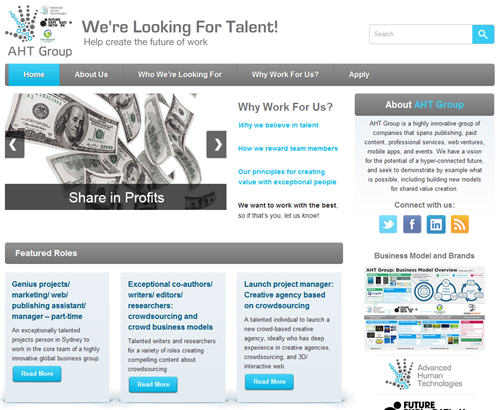**Screenshot of A.H.T. Group Web Page**

The screenshot depicts a web page from A.H.T. Group, viewed on a desktop or laptop browser. At the very top, the company's logo—a hand composed of various sized dots in light gray and bright light blue—captures attention. To the logo's right, a tagline reads, "We're Looking for Talent, Help Create the Future of Work."

The web page's color scheme is predominantly white, bright light blue, and light to medium gray. The light to medium gray is prominently used for the headers and menu backgrounds, with white text within these gray sections. The main body of the text is displayed in light gray, while titles stand out in bright blue, ensuring easy readability.

Below the header, the main menu contains text-based navigation options: Home, About Us, We're Looking for You, Why Work for Us, and Apply. To the right of the menu, a search bar allows for easy content discovery on the site.

Further down the page, multiple paragraphs of information are presented. A dynamic image depicting $100 bills featuring Benjamin Franklin being thrown into the air and falling adds a visual element to the text content, emphasizing financial success or prosperity. These are clearly U.S. dollars.

Four distinct social media icons—Twitter, Facebook, Indeed, and an RSS feed symbolized by a yellow icon with a Wi-Fi symbol—are also displayed, suggesting the company's presence on these platforms.

Overall, the web page design combines clean aesthetics with functional navigation, aiming to attract talent and provide a clear pathway for users to engage with the company.